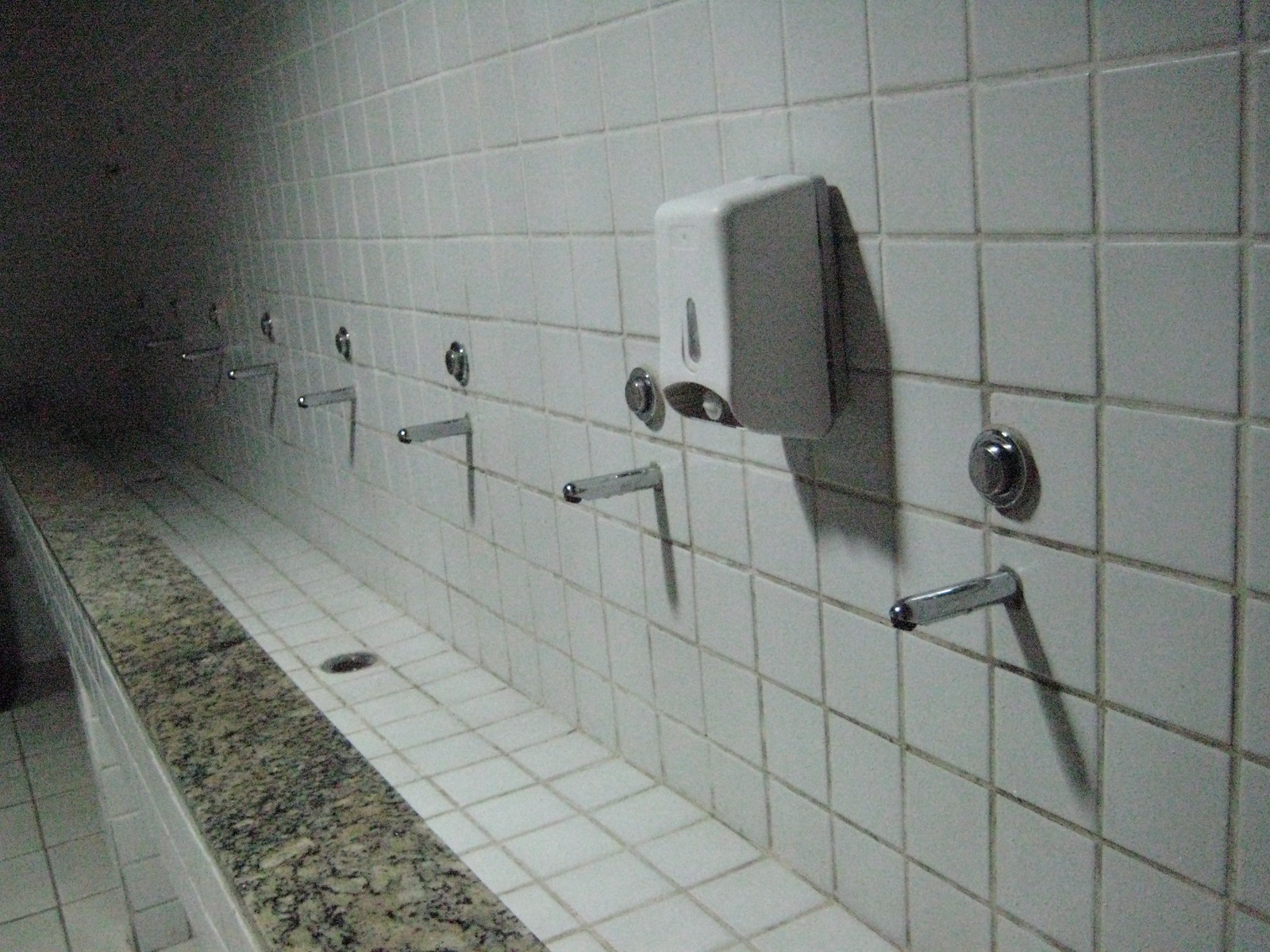This is a photograph of a dimly-lit bathroom featuring a long, narrow, hand-washing trough. The whole room is adorned in ceramic white square tiles that cover the walls, floor, and the sink section. The trough-like sink has several metal faucets mounted on the tiled wall, each equipped with an activation button situated above. Notably, a white plastic soap dispenser with a gray backing is affixed to the wall between a couple of these faucets. The marble-finished strip edging the sink adds a touch of contrast to the predominantly ceramic setup. The sink also includes a drain in the middle, and one visible post, covered in the same white tiles, supports the structure. The overall atmosphere of the bathroom is quite dreary due to the poor lighting.